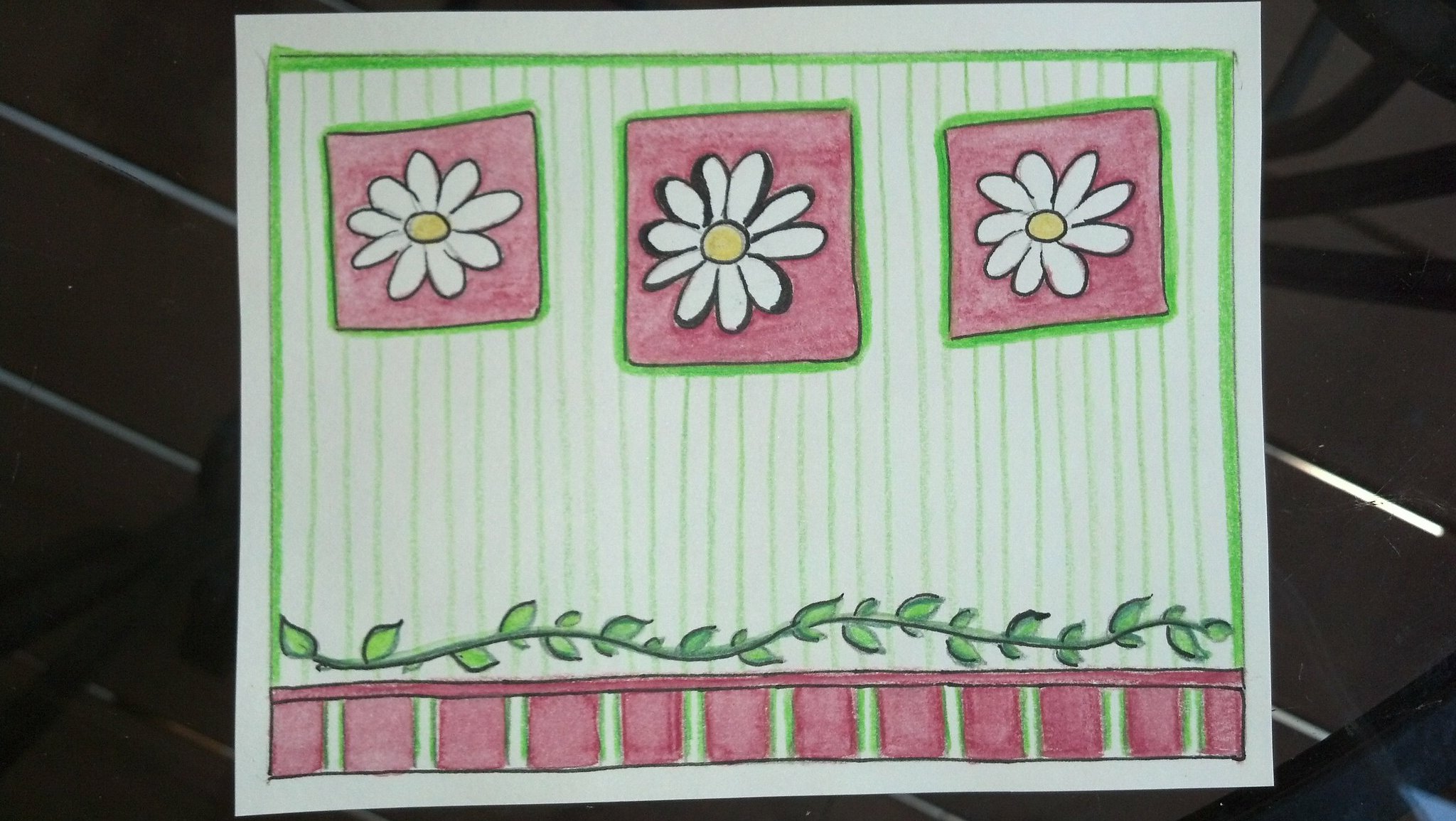This photograph captures an artistic drawing on a white sheet of cardstock or possibly sketchbook or printer paper. The top section of the drawing features several red tiles adorned with intricately detailed white daisies at their centers, all highlighted by green outlines. These tiles are set against what seems to be a striped green backdrop, giving the impression of either a wall or a fence.

Beneath this tiled section runs a wavy, elongated vine adorned with small leaves on both sides, adding a dynamic, natural element to the composition. Below this vine is a distinct border that could either represent another fence or a flowerbed. This border is composed of alternating red and green stripes, with the red stripes being noticeably thicker.

The entire drawing is positioned on a dark gray background, providing a stark contrast that accentuates the vibrant colors and intricate details of the artwork.